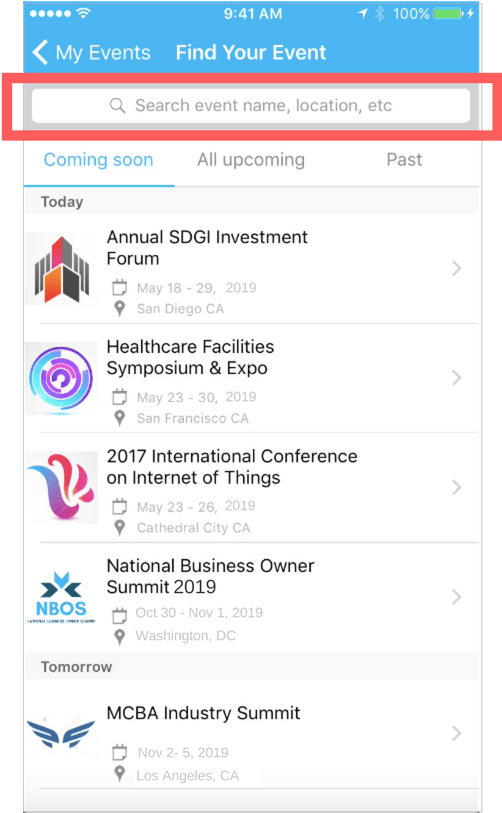Sure, here’s a cleaned-up and detailed caption for the image described:

---

Screenshot of a mobile view from an event website taken at 9:41 AM with full battery and signal strength. The top section has a light blue background with icons for connectivity and battery life. Below that, the page header reads "Find Your Event," flanked by a back arrow labeled "My Events" on the left. A search bar with placeholder text "Search event name, location, etc." is prominently featured.

Beneath the search bar, there are three navigational options: "Coming Soon" highlighted in blue, "All Upcoming" and "Past" in grey. Currently selected is "Coming Soon." The main content begins with "Today," listing events with associated symbols.

1. **Annual SDGI Investment Forum**
   - Date: May 18th - 29th, 2019 (greyed out)
   - Location: San Diego, California

2. **Healthcare Facility Symposium and Expo**
   - Date: May 23rd - 30th, 2019 (greyed out)
   - Location: San Francisco, California

3. **2017 International Conference on Internet of Things**
   - Date: May 23rd - 26th, 2019 (greyed out)
   - Location: Cathedral City, California

4. **National Business Owner Summit 2019**
   - Date: October 30th - November 1st, 2019 (greyed out)
   - Location: Washington, D.C.

The section labeled "Tomorrow" features one event:
- **MCBA Industry Summit**
  - Date: November 2nd - 5th, 2019 (greyed out)
  - Location: Los Angeles, California
  - Symbol: Blue wings

---